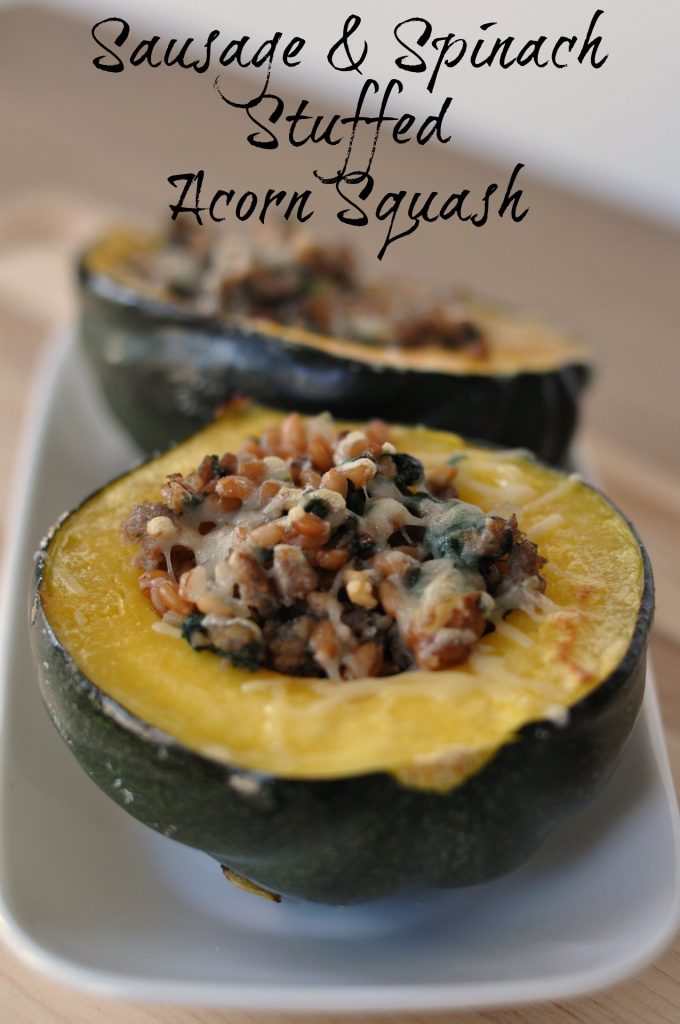The image features two halves of a round, acorn squash, cut and positioned with the cut side facing upward on a white rectangular dish that is placed on a table top. Each half of the dark green-skinned squash is generously stuffed with a mixture containing sausage, spinach, corn, tomato, rice or lentils, and topped with melted, shredded white cheese. The stuffing displays a variety of colors and textures: brown sausage, green spinach, yellow corn, and small round objects likely to be rice or lentils. The front half of the squash is in clear focus, while the second half begins to fade into the background. Above the dish, the caption "Sausage & Spinach Stuffed Acorn Squash" is elegantly written in black, cursive lettering, akin to a fountain pen's handwriting.